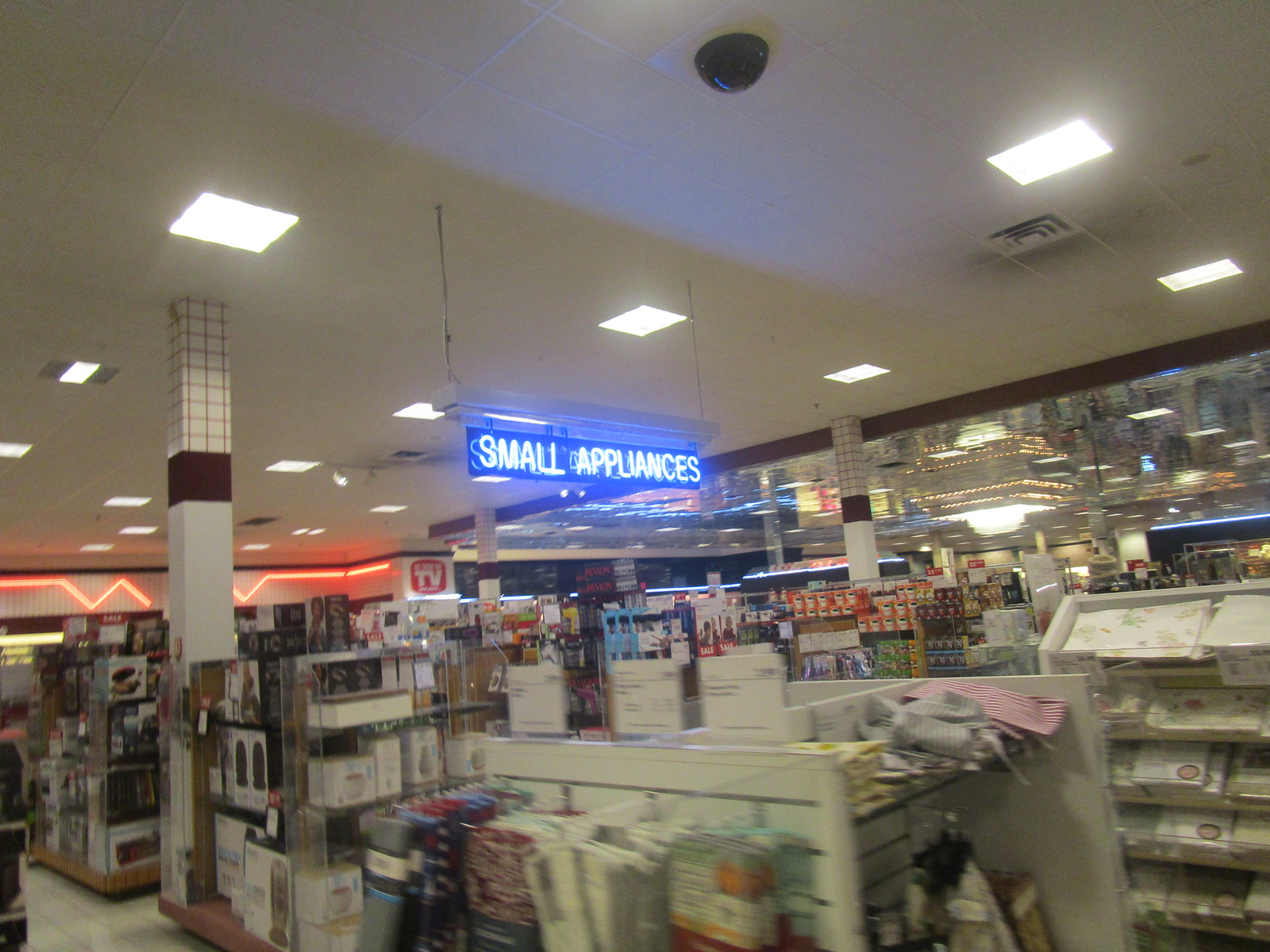This color photograph captures the interior of a spacious, somewhat dated retail store. The ceiling, adorned with white square fluorescent lights and an air conditioning register, features a black circular dome for a security camera. Prominently hanging from the ceiling in the center of the image is a rectangular blue neon sign that reads "Small Appliances." The store's aisles are visible, with the closest in the foreground displaying shelves stocked with towels. The blurred quality of the photo makes the aisle signs difficult to read, but the home goods section is discernible with items like placemats, sheets, cloth napkins, and aprons. Support pillars stretch from floor to ceiling, some clad in tile that hints at decor from the 80s or 90s. In the background, a red zigzagging neon light decorates the back wall, alongside a sign labeled "As Seen on TV." The store appears empty of people.